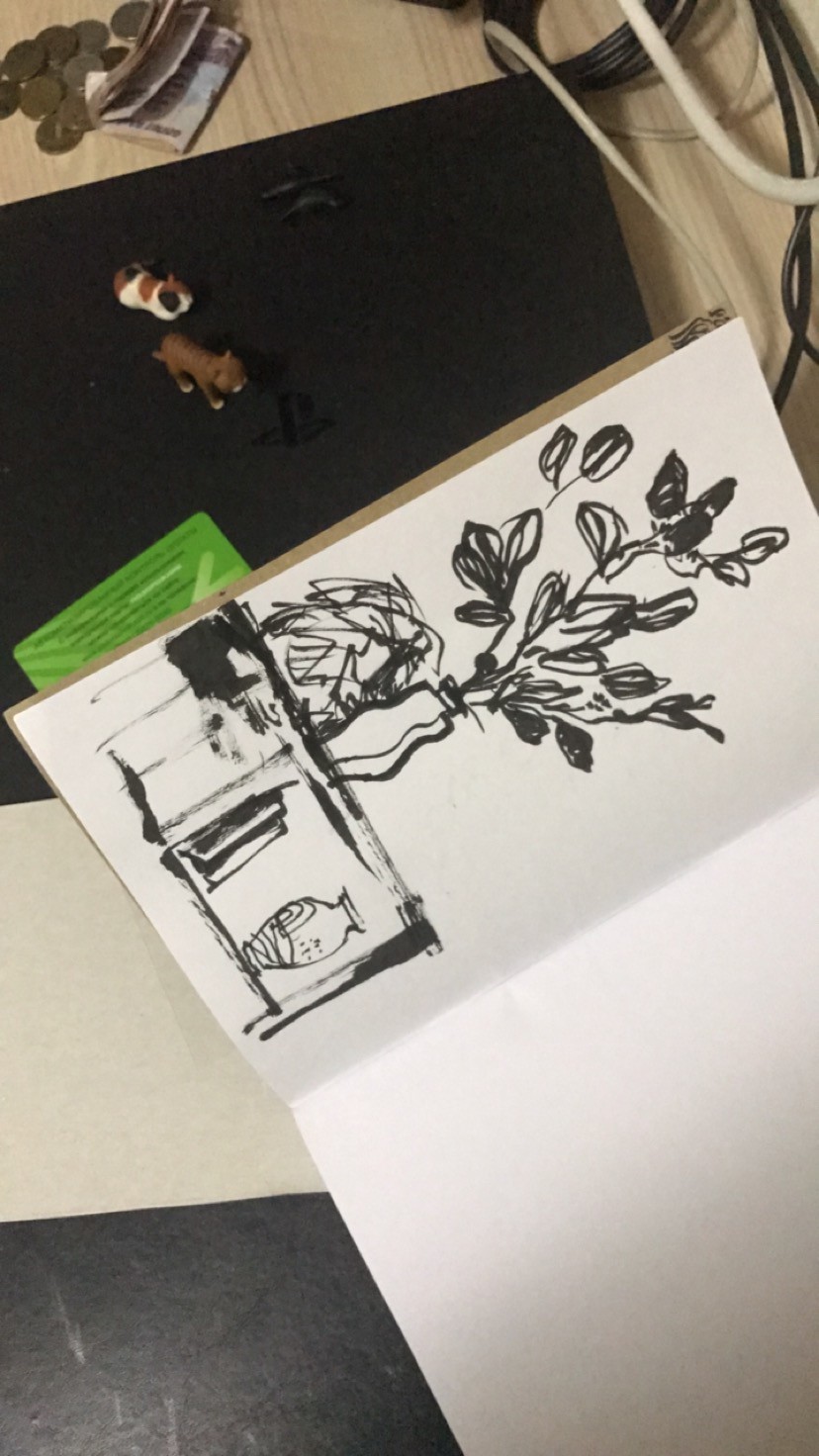In this photograph, a white notebook is prominently featured, displaying a black ink hand-drawn illustration of a table. The table is depicted with a vase containing leaves and flowers atop it, and another vase situated on a shelf beneath the table surface. Positioned behind the notebook, a green object resembling a bus pass or credit card is noticeable. To the right-hand side, the upper corner is cluttered with a jumble of electrical cords. The entire scene rests on a sleek black desk. Adding a whimsical touch, two small plastic cat figurines are placed on the desk. Just above these figurines, a small pile of coins and some folded dollar bills can be seen, completing the tableau.